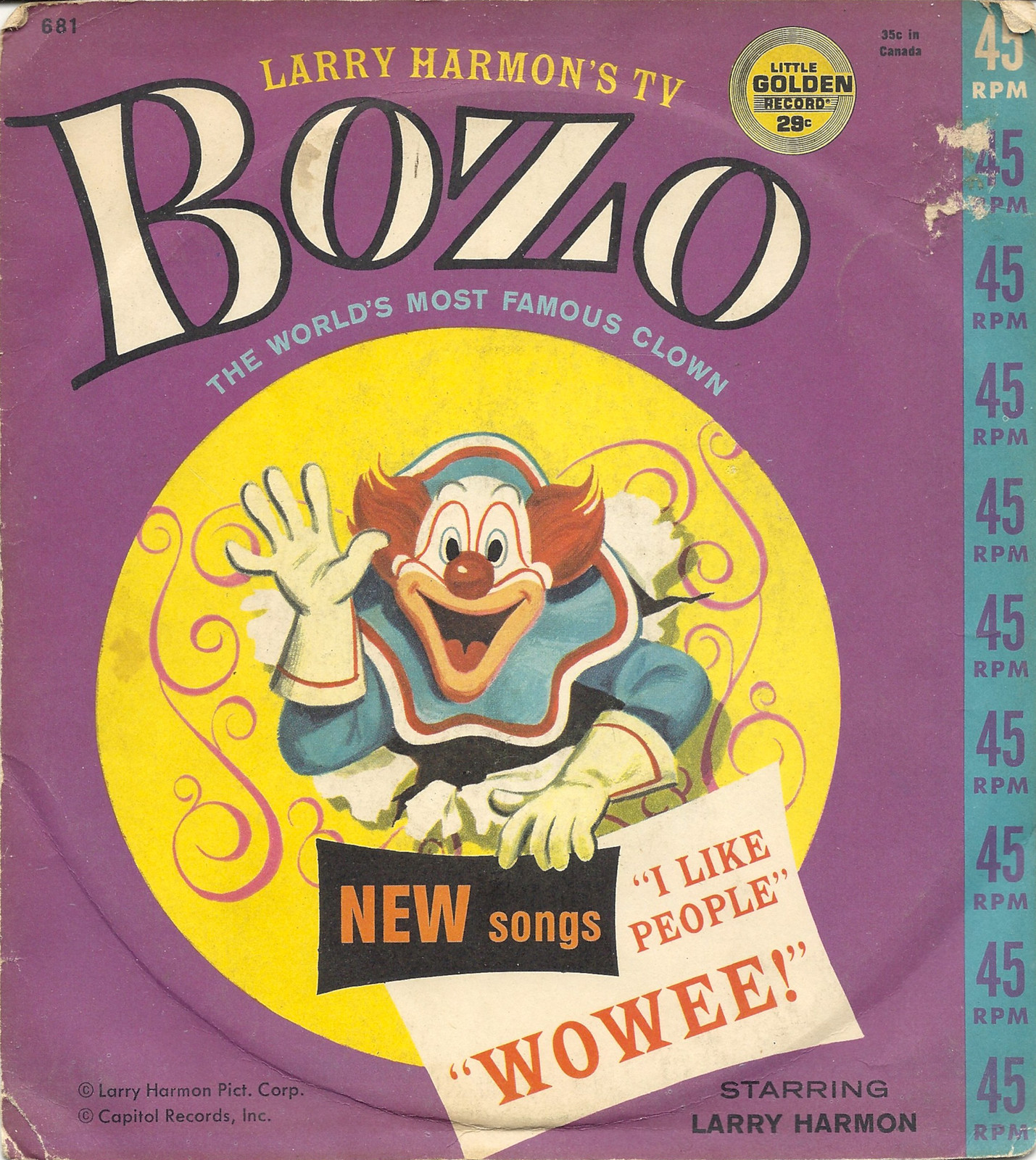This image is a detailed scan of a classic 45 RPM vinyl record cover from the 1960s or 70s, featuring Bozo the Clown, voiced by Larry Harmon. The cover showcases a vibrant light purple background with a distinctive blue vertical strip on the right side, repeatedly marked with "45 RPM". Prominently displayed in white text with a dark border at the top is "Bozo," followed by "The World's Most Famous Clown" in blue. Central to the design is a yellow circle adorned with flowery ornamentation, inside which Bozo is depicted with iconic white face paint, a big red nose, and red hair. Bozo is shown with a big smile, raised right hand, and waving while wearing red gloves and a blue clown outfit with red and white stripes. He holds two signs: a smaller dark rectangular one reading "New Songs" in red, and a larger rectangular one below stating "I Like People". Additional information at the bottom left mentions the Larry Harmon Picture Corporation and Capitol Records Incorporated. The cover nostalgically reflects its time, evoking memories of when such records were sold for 35 cents in Canada and 29 cents in the U.S. as part of Little Golden Records, often including storybooks for children.